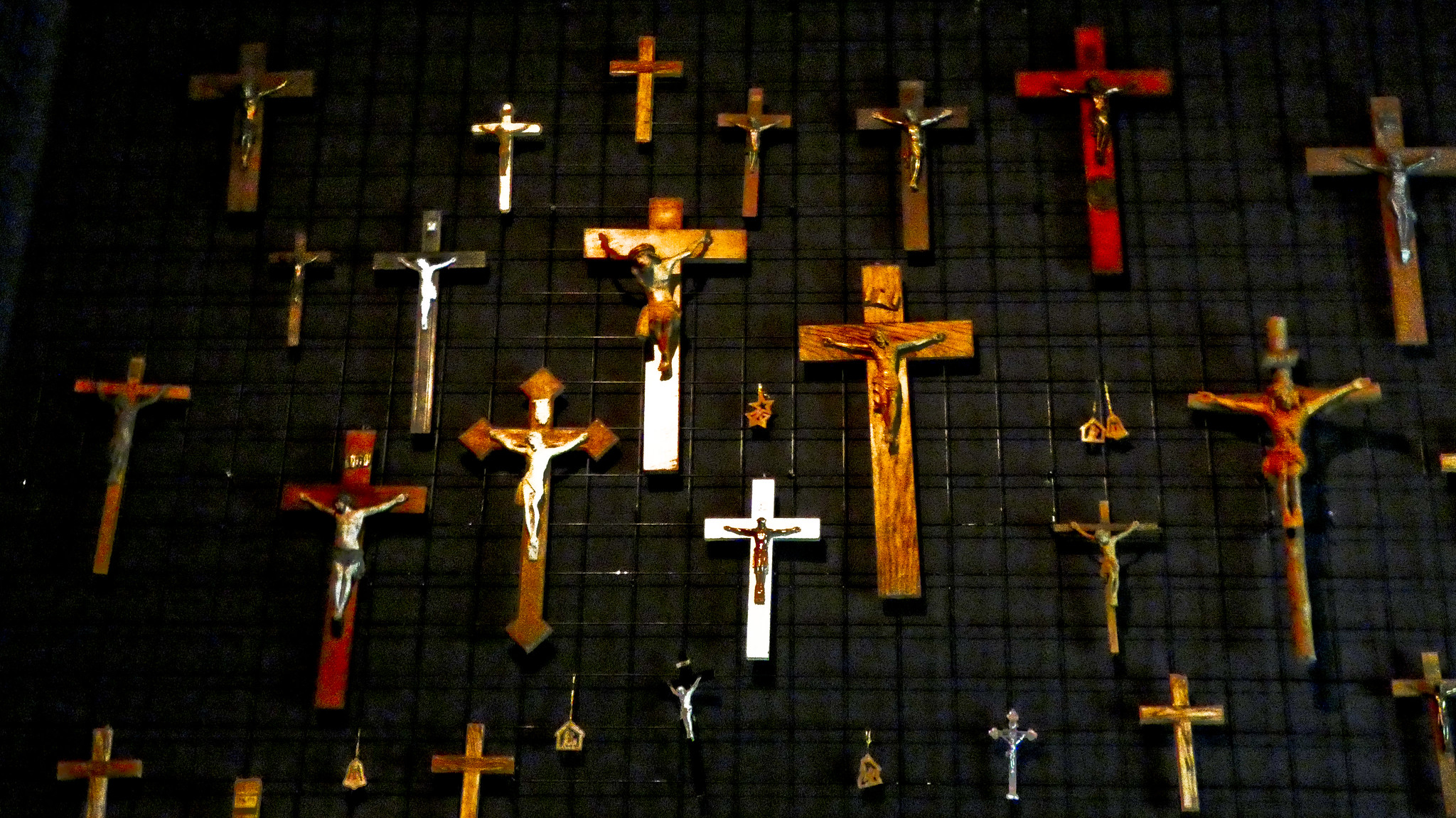This is a detailed colour photograph, possibly AI-generated art, featuring an array of crucifixes and other small wooden objects, all hanging against a black background adorned with a square embossed pattern. The glossy surface of the background catches glimpses of light, enhancing the overall visual effect. The crucifixes, mostly wooden and varying in shapes and sizes, are illuminated and meticulously aligned from top to bottom. Each crucifix primarily follows the Catholic design, with almost all featuring the figure of Jesus. The central crucifix is particularly striking, being almost white at the bottom with a small light at the top, making it the most illuminated and in focus. 

The crosses come in various colours and materials: predominantly wooden, with some in red, silver, gold, and combinations where the figure of Jesus and the cross differ in colour. Among the myriad of crucifixes, there are a few smaller, plain wooden crosses and other tiny illuminated ornaments, one of which appears to be silver and resembles a small manger scene. A noticeable wire grid or chain-like structure supports these items, casting subtle shadows on the backdrop. Some crosses also feature unique embellishments, such as round sticks and diamond-shaped ends, contributing to the intricate diversity of this captivating display.